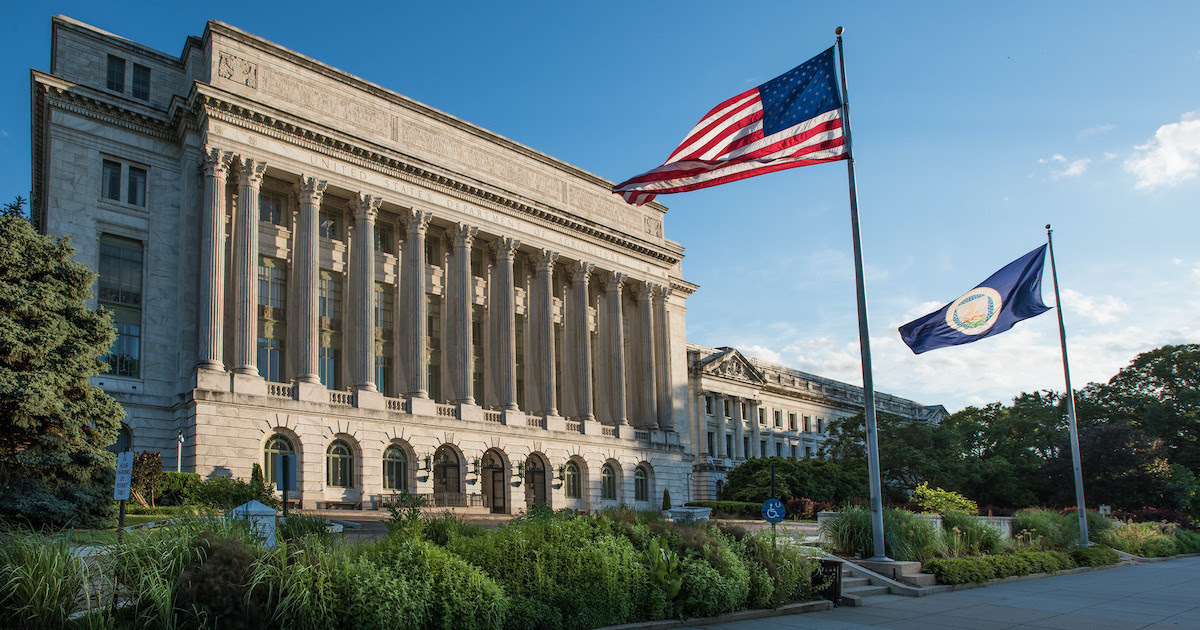This photograph captures the majestic exterior of a large, stately building, presumably a government or state building, constructed from stone or white concrete. The imposing structure features tall columns spanning the upper level across the front facade, and a series of elegant arched windows and doorways on the ground floor, adding to its grandeur. Dominating the foreground is a neatly landscaped area flanking a broad concrete stairwell that ascends to the building's entrance. Prominently positioned within the landscaping are two flagpoles: the taller one bearing the American flag, which flows gracefully to the left, and a shorter pole flying a blue flag, likely representing a state or official entity. In the background, another masonry building is partially visible, extending the sense of an expansive civic complex. The scene is set under a clear blue sky dotted with wispy white clouds, with trees providing a natural backdrop.